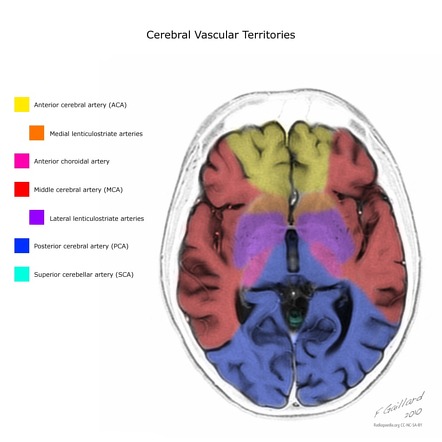The image is a detailed infographic of the human brain viewed from the top, presenting the Cerebrovascular Territories with transparent scalp boundaries. On the right, the brain is segmented and color-coded to indicate different vascular regions, while the left side features corresponding labels. At the top, the image is titled "Cerebrovascular Territories." The sections are labeled from yellow to green, starting with the Anterior Cerebral Artery (ACA) in yellow at the top part of the brain. Below the yellow section is the purple area labeled as the Lateral Lenticulostriate Artery, followed by the blue area below it. The side of the brain shows the pink Anterior Choroidal Artery. The red section represents the Middle Cerebral Artery, and the orange Medial Lenticulostriate Arteries are indicated. The artist, F. Gaylord, has meticulously illustrated these regions with clear demarcations and vibrant colors for educational purposes.